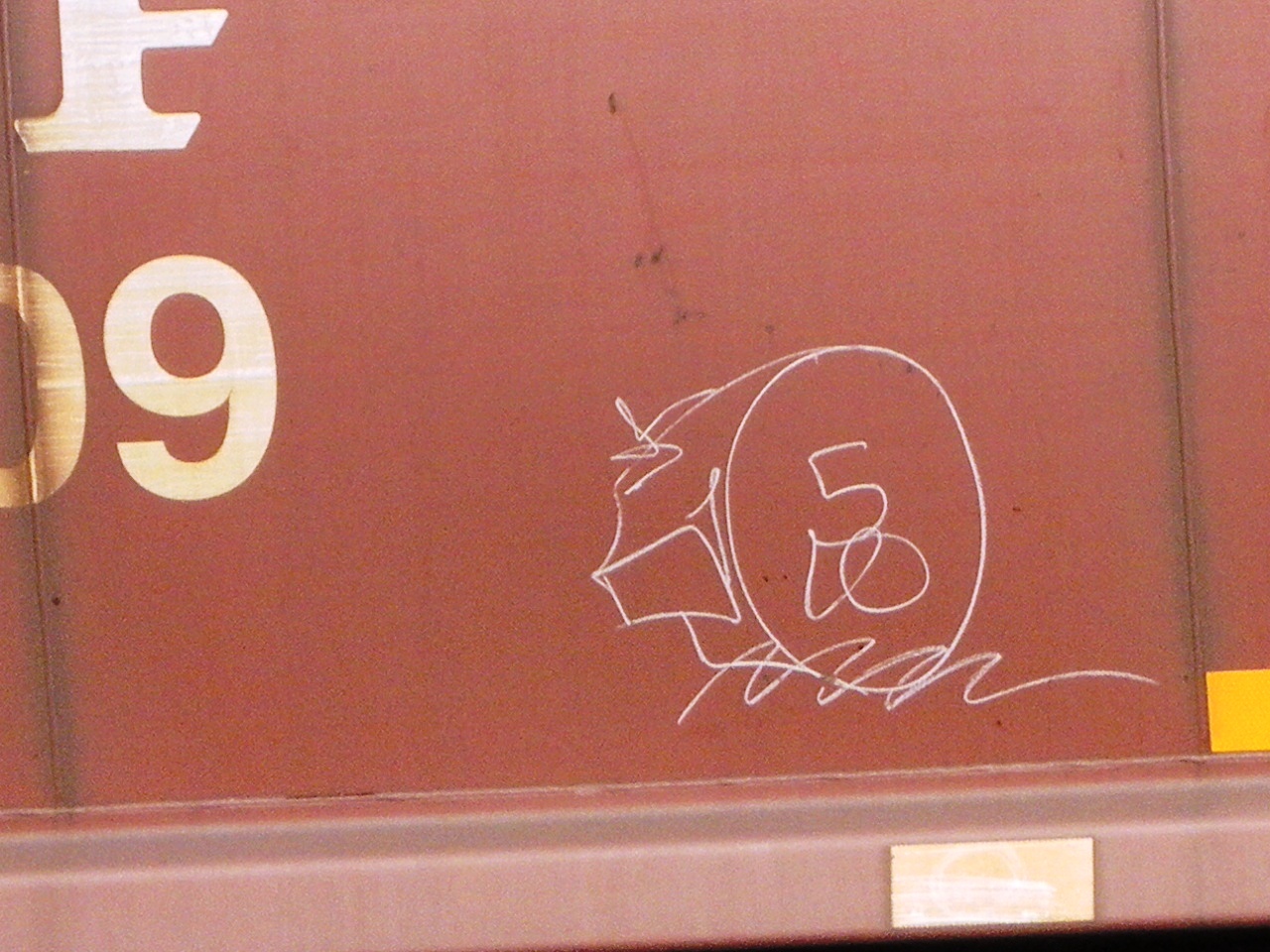This detailed photo showcases the rear of a red emergency vehicle, likely a fire truck, prominently marked by distinguishing features. In the top left corner, the vehicle displays the letter 'F' and the number '09' painted in gold. At the bottom, a red metal bumper bar is present, adorned with two yellow stickers. An intricate piece of white graffiti dominates the image, located in the bottom left corner. The graffiti resembles a whistle, encircling the number '50' and accompanied by swirling lines and an unknown signature. Additional yellow striping enhances the bottom section of the vehicle, adding contrast to the overall red background.